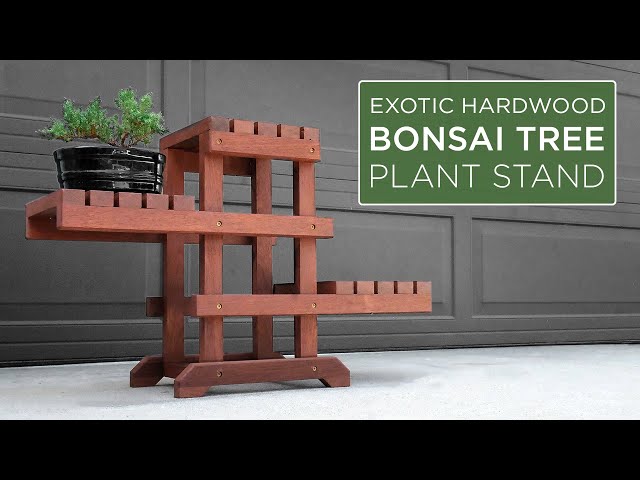The image is a rectangular-shaped photograph with the longer sides stretching from left to right, framed by a black border at the top and bottom. It prominently features a bonsai tree stand, which is positioned towards the right side of the image. The stand itself is crafted from what appears to be redwood or another dark wood and is structured in three tiers. To its right, a conspicuous label or sign bordered in white showcases a green background with white text. The text on the label reads "Exotic Hardwood Bonsai Tree Plant Stand," with the words "Bonsai Tree" emphasized in bold, while "Plant Stand" appears in a larger font but not bolded. The ground beneath the stand is white and offers a stark contrast to the rich hues of the wooden structure. On the left side of the bonsai tree stand rests a single plant, drawing attention to the stand's utilitarian function and aesthetic appeal.